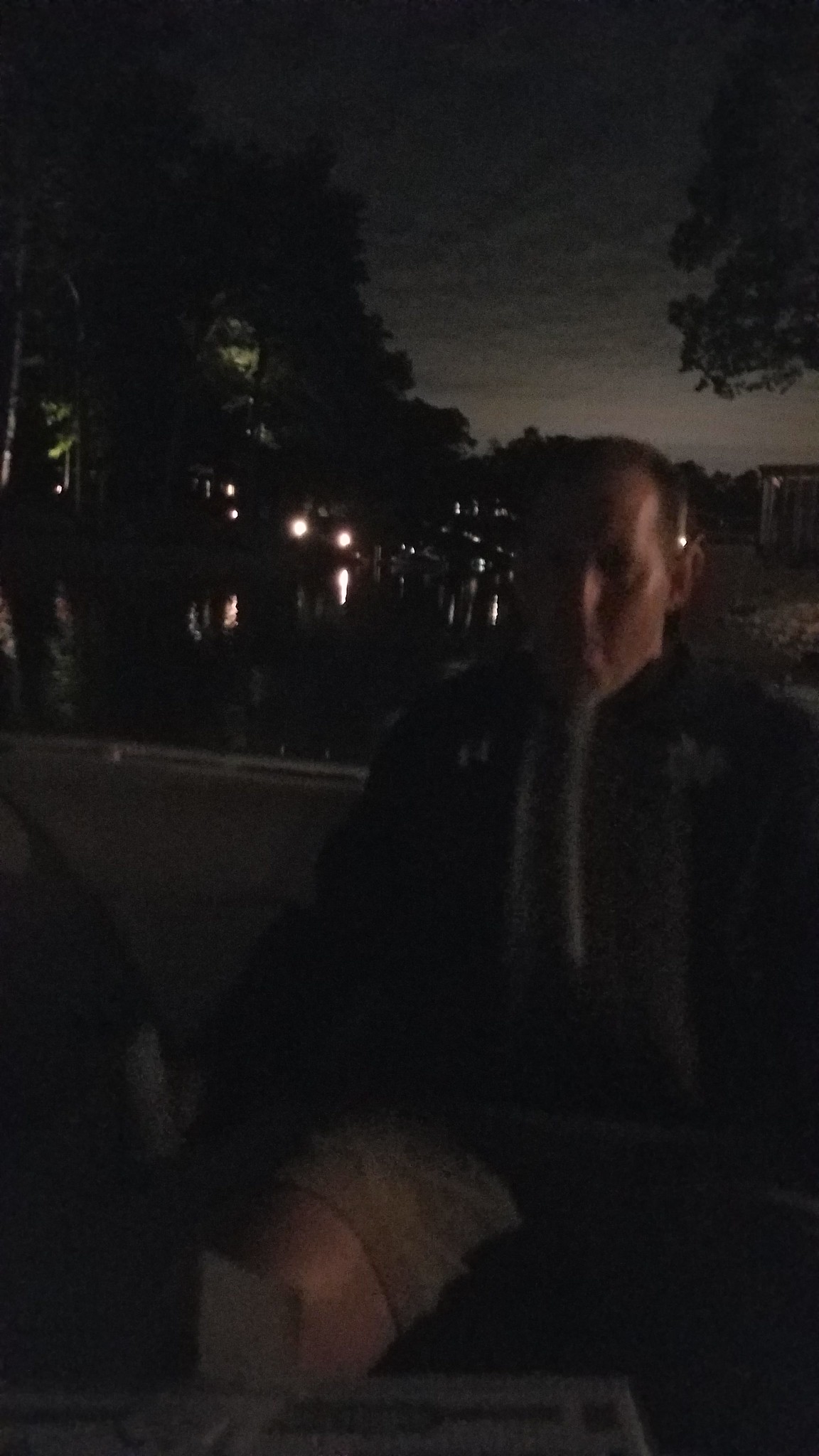In the dim light of dusk, a man stands outdoors, silhouetted against a dramatic evening sky marked by dark clouds transitioning to lighter grays near the horizon, hinting at the setting sun. He is dressed in a sweater adorned with long, grayish tassels that sway slightly in the evening breeze. Cradled in his arms is a curious object with a brown base, seemingly filled with hay. Closer to the camera, at the very bottom of the image, a box sits, its contents obscured by shadows. To the left, the dark outlines of trees add to the moodiness of the scene, while scattered lights from vehicles or possibly distant houses twinkle in the background. These lights create shimmering reflections on a nearby river or lake, adding a touch of enchantment to the twilight atmosphere.